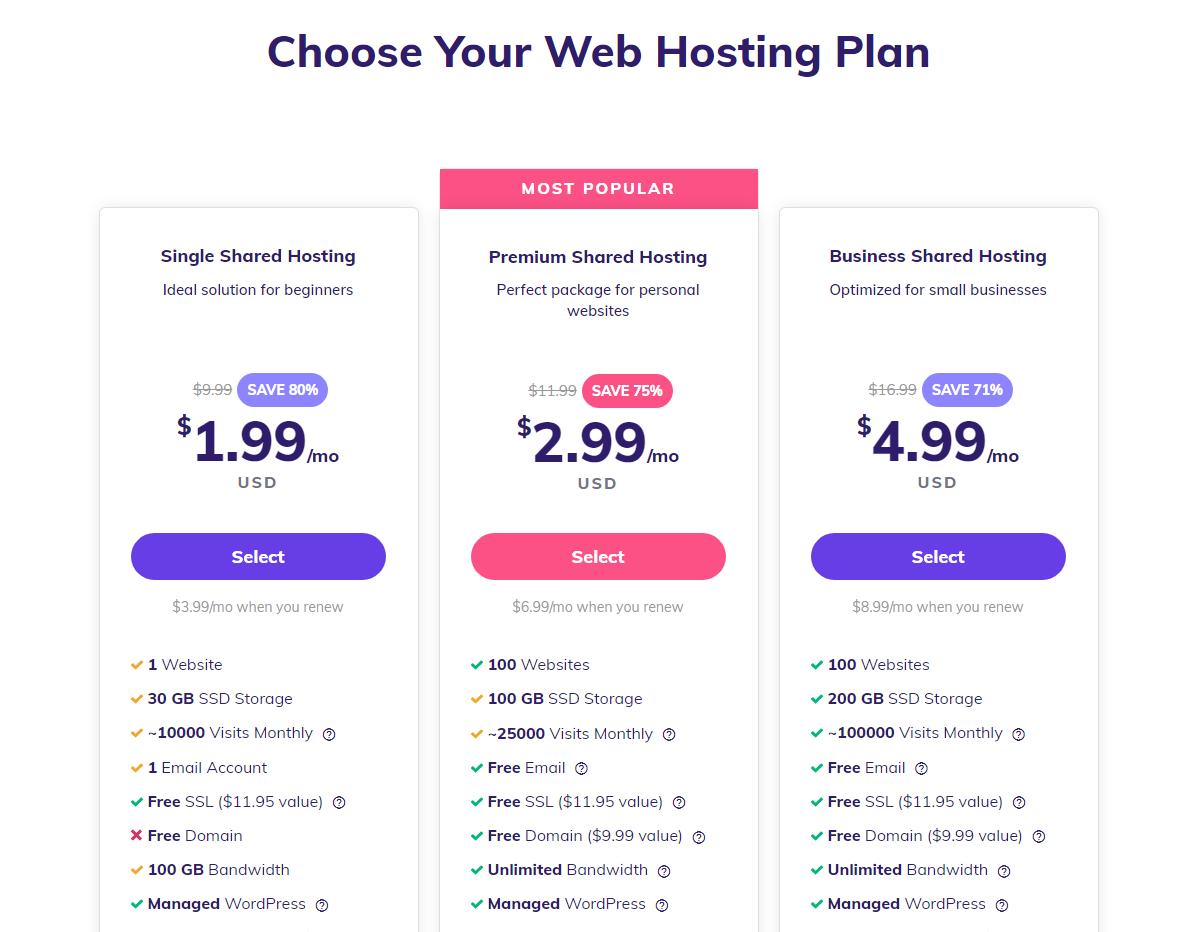The screenshot is of a web page showcasing various web hosting plans. At the top of the page, the text "Choose Your Web Hosting Plan" is prominently displayed. In the lower-central area of the image, there are three vertically aligned rectangles, each representing a different hosting plan with detailed information.

1. **Single Shared Hosting (Left Plan):**
   This plan is described as the "Ideal Solution for Beginners." Originally priced at $9.99, the cost is now reduced to $1.99 per month (USD), an 80% savings, highlighted next to the original price. There is an option to "Select" this plan. Note that the renewal rate for this plan is $3.99 per month. The features for this plan include:
   - Host one website
   - 30 GB SSD storage
   - Supports up to 10,000 monthly visitors
   - One email account
   - Free SSL certificate (valued at $11.95)
   - Free domain
   - 1 GB bandwidth
   - Managed WordPress

2. **Premium Shared Hosting (Center Plan):**
   Marked as the "Most Popular" option, with this label displayed in a red rectangle above the plan's name. This plan is called the "Perfect Package for Personal Websites" and is priced at $2.99 per month. A button to "Select" this plan is present, and the same detailed feature list provided below follows a similar structure.

3. **Business Shared Hosting (Right Plan):**
   This plan is designed for business use and is priced at $4.99 per month. Like the other plans, this has a "Select" button and an accompanying list of features, although the specific features are not detailed in the provided text. 

The image layout clearly delineates each web hosting plan's details, ensuring easy comparison, with the offers and features prominently displayed for potential customers.